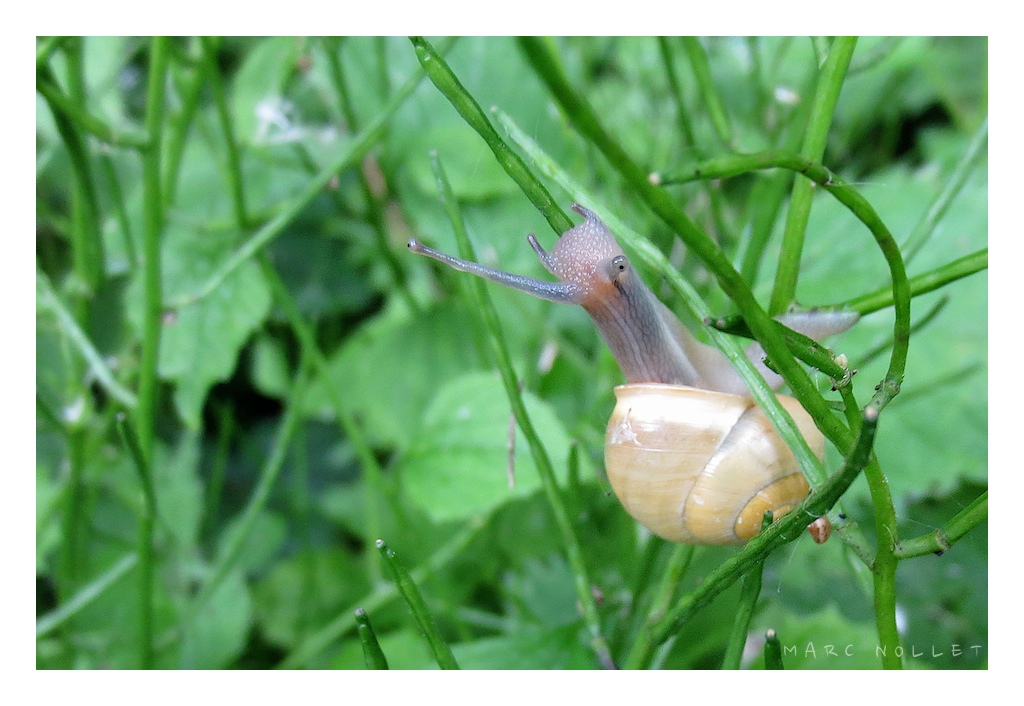This detailed close-up photograph, taken by Mark Nolet, captures the intricate beauty of a snail crawling on vibrant greenery. Dominating almost half of the image, the snail is climbing along a green stalk, surrounded by an abundance of plant stems and large leaves that make up the lush background. The snail's pearlescent, off-white tan shell displays a captivating spiral pattern. Its semi-translucent skin reveals subtle hues of gray, black, and red, adding to the visual complexity. The snail's head and neck are stretched out, showcasing its antennae and feelers in striking detail. Sunlight filters through the leaves, illuminating the scene and highlighting the natural colors of green, tan, brown, and the snail's pearlescent shell. Near the bottom right corner, the photographer's signature "Mark Nolet" is elegantly displayed in white font.